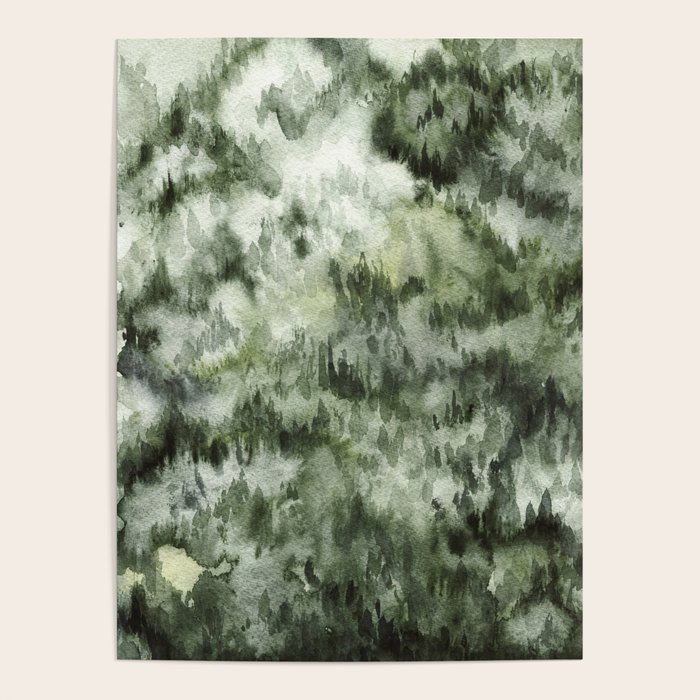The image portrays an abstract watercolor painting on an A5-sized canvas mounted on a uniform gray wall. Dominated by various shades of green, from deep forest greens to lighter, more foraged hues, the artwork uses consistent brushstrokes to create a sense of depth and space. The dark and light green tones are accented with hints of black and gray, culminating in patterns that evoke the dense, layered foliage of a forest with numerous treetops. The painter has skillfully used splotches and shaded areas, particularly darkening the top right corner, to indicate spacing and depth among the trees, adding to the abstract yet nature-inspired essence of the piece. There is no text on the painting, emphasizing the visual elements and textures that convey a serene, mysterious woodland scene.